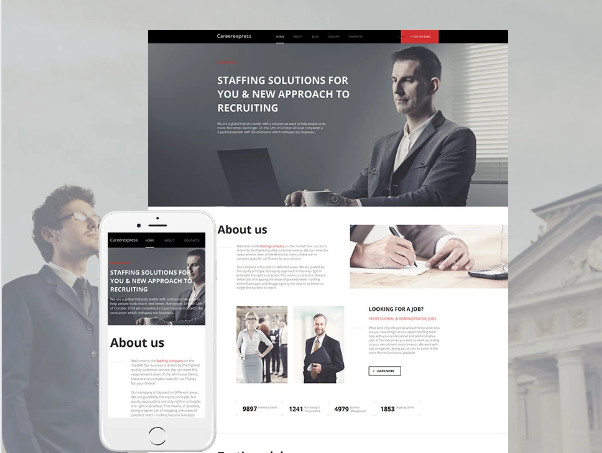A highly detailed web page showcases a multifaceted recruitment platform. The background prominently features an older gentleman reminiscent of Leon Trotsky, gazing skyward, reminiscent of historical revolutionary imagery. On the right side of the screen stands an imposing courthouse-like building, adding a touch of gravitas to the scene.

In the foreground, overlaid projections create a dynamic interface. At the top, a black band accented with a small red bar presents a hard-to-read message beside a man in a suit—tie-less, diligently working on his laptop. A steaming cup of coffee sits beside him, emphasizing a modern, professional environment. Bold white letters proclaim, "Staffing Solutions for You" and "A New Approach to Recruiting."

Below this heading is a paragraph, obscured by a digital rendering of a smartphone showcasing the same app interface. The screen reads "About Us," accompanied by several unreadable paragraphs, likely detailing the company's ethos and services. Adjacent to this, multiple images display satisfied clients or job-seekers, adding a human touch to the corporate narrative.

To the right, a prominent image of an individual completing an application form is labeled "Looking for a Job." Below this image is a call-to-action button, encouraging users to initiate their job search. This web layout effectively bridges the gap between employers and job-seekers, enticing both parties with an intuitive, engaging design.